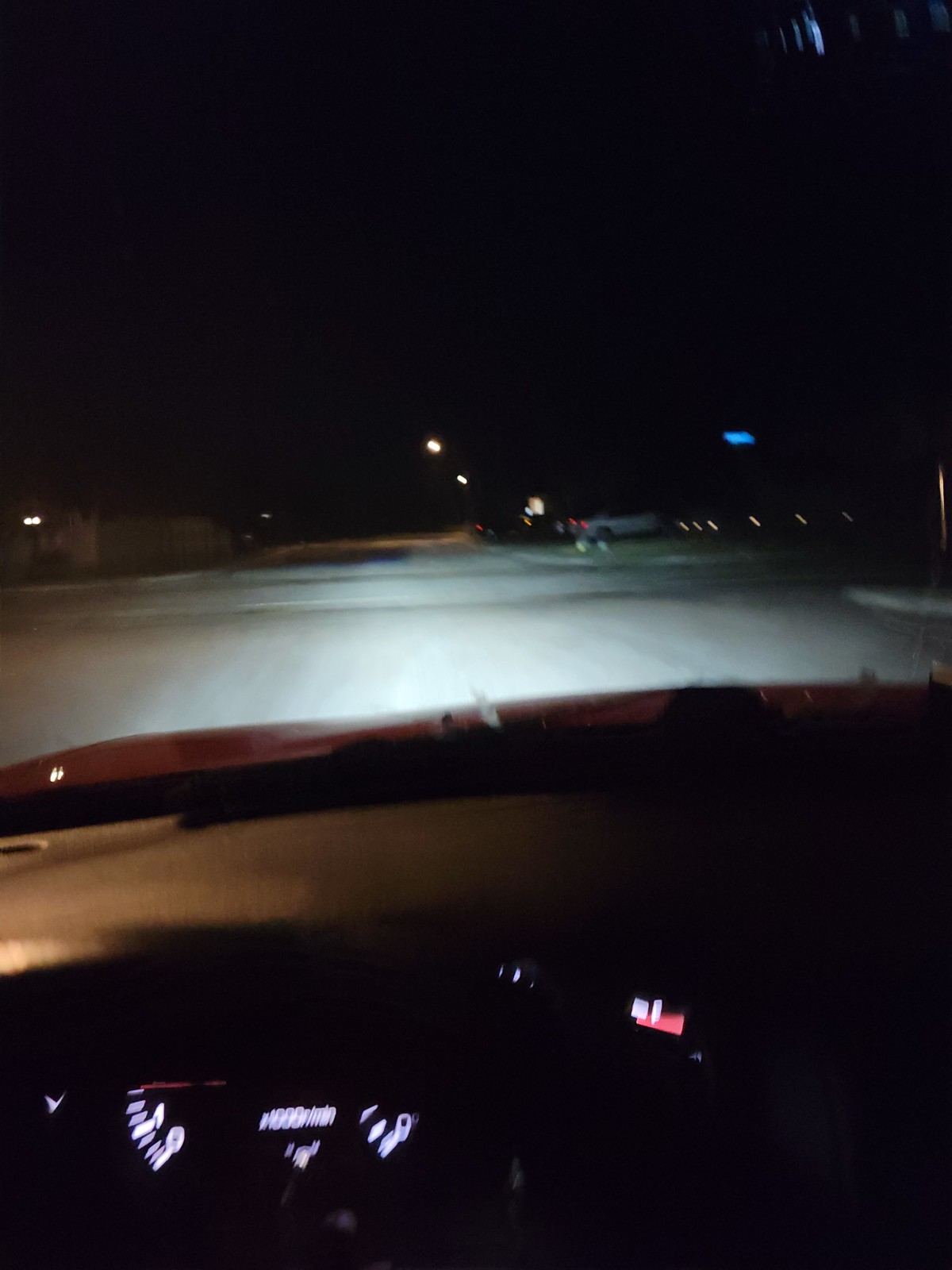Captured from the interior of a moving car, this image presents an engaging composition of both the vehicle's dashboard and the street ahead. The black dashboard anchors the foreground, with the windshield wipers faintly visible outside. Intriguing shadows play across the top part of the image, hinting at a window. The control panel on the dash is partially illuminated, showcasing various indicators, including a blurred speedometer with glowing white lights. The faint outline of a steering wheel is discernible, adding to the authentic feel of the scene.

To the right of the speedometer, additional dashboard lights emerge, featuring a small red light accompanied by white markings, possibly indicating fuel or oil levels. Extending beyond the car's interior, the light gray road stretches forward under a dark sky. Illuminated streetlights line the right side, where a car is seemingly parked in a nearby lot. A small, lit blue sign suggests a store in the background. On the left side of the road, some indistinct buildings contribute to the urban ambiance. The car's headlights cast a sheen on the pavement, emphasizing the nocturnal setting and lending a sense of movement to the otherwise tranquil scene.